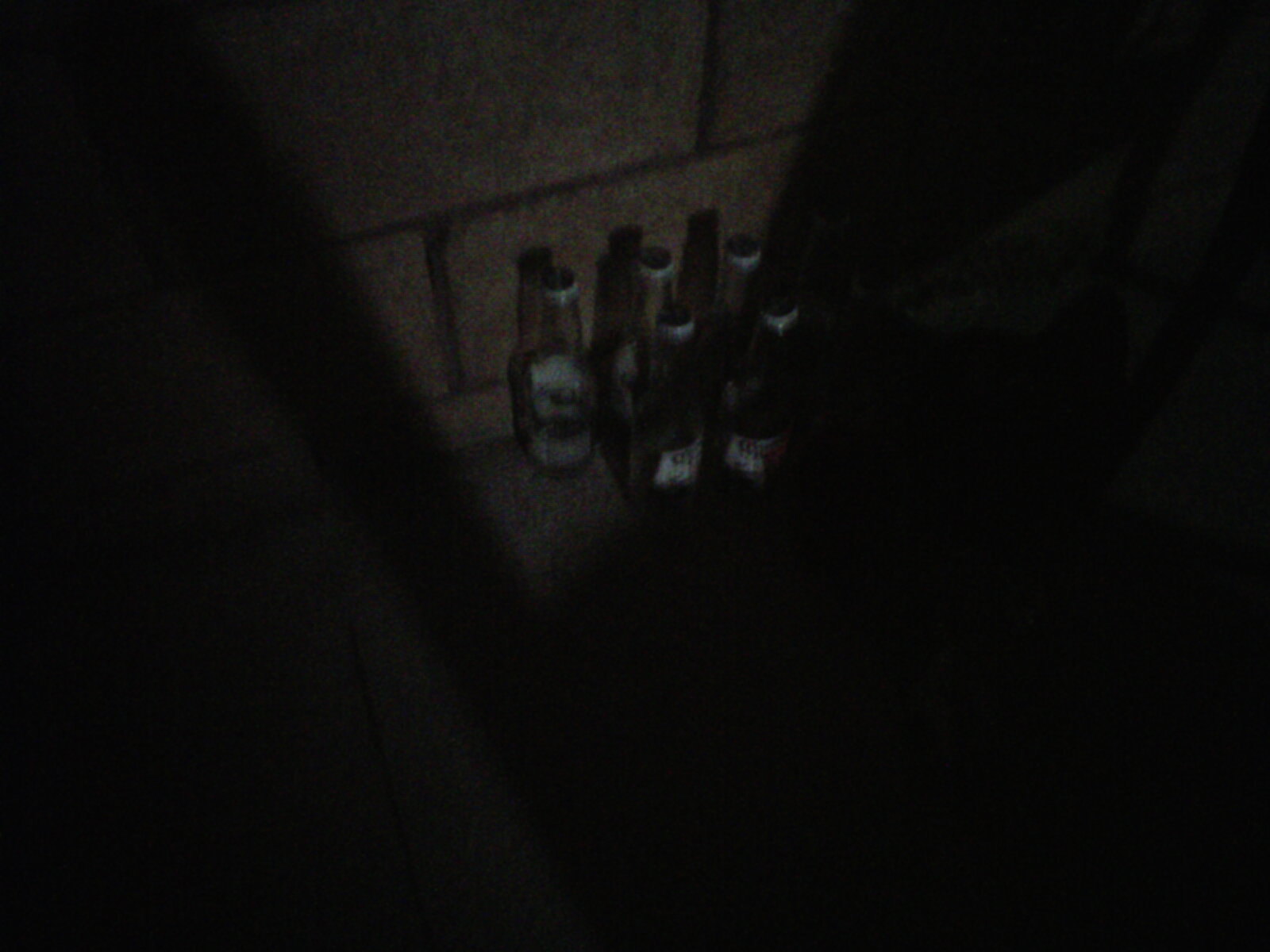In this dark, nighttime urban outdoor photograph, five empty glass bottles are positioned on a sidewalk against a concrete block wall with dark grout. The bottles, which appear to be either wine or beer, are arranged with three at the back directly against the wall and two in front of them. The labels on the bottles are faintly visible but unreadable in the poor lighting, likely white or a light color. Each bottle is sealed with a top or cork, suggesting they were resealed after being emptied. The photograph captures minimal detail due to the lack of available light, casting most of the surroundings in shadows and leaving only the arrangement of the bottles and part of the wall discernible.